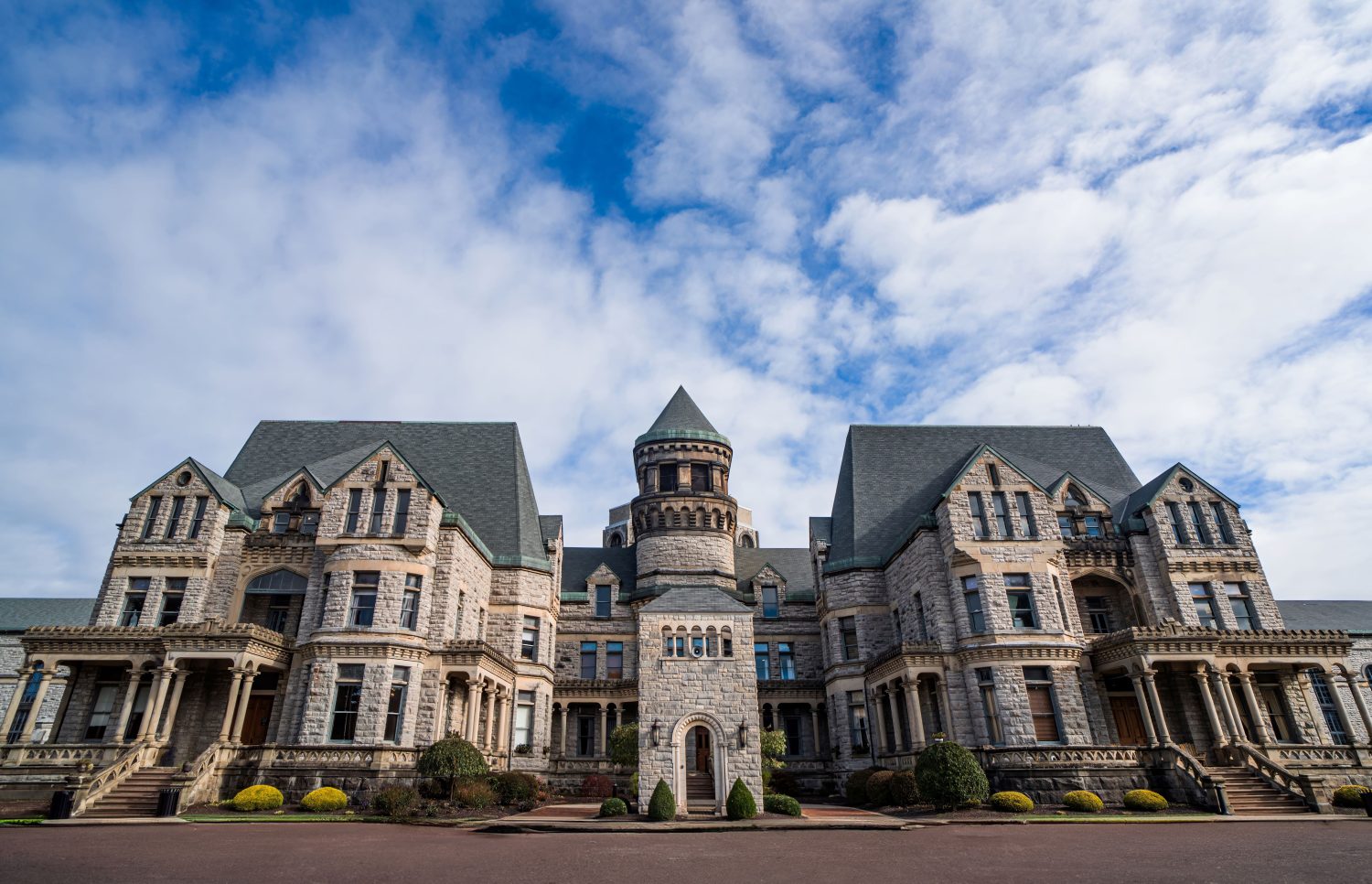The image showcases the front view of an enormous, symmetrical mansion built from light gray bricks, resembling both a grand home and a small castle. The mansion appears to have three stories, with three rows of windows uniformly spread across both sides. Each side of the house is mirror-like, featuring identical facades connected by a central tower adorned with a pointed, cathedral-esque roof. The structure's roofing exhibits a dark gray or bluish tint, enhancing its grandeur.

At the base of the mansion, there is a considerable amount of shrubbery that adds to the lush appearance of the property. Each identical section of the mansion houses separate entrances, each accessible via small staircases leading up to stately brown doors. These entrances are complemented by cozy porches. Directly in front of the house, a light brown or light purple driveway is visible, with its texture blending into the surrounding landscaping.

The top part of the mansion, including the main tower, exhibits a subtle grayish-green hue, furthering the structure's historical and majestic aesthetic. Above the mansion, the sky forms a captivating backdrop, filled with a mix of white clouds and patches of clear blue. The overall impression given is one of architectural splendor, heightened by the grand size and detailed symmetry of the mansion.